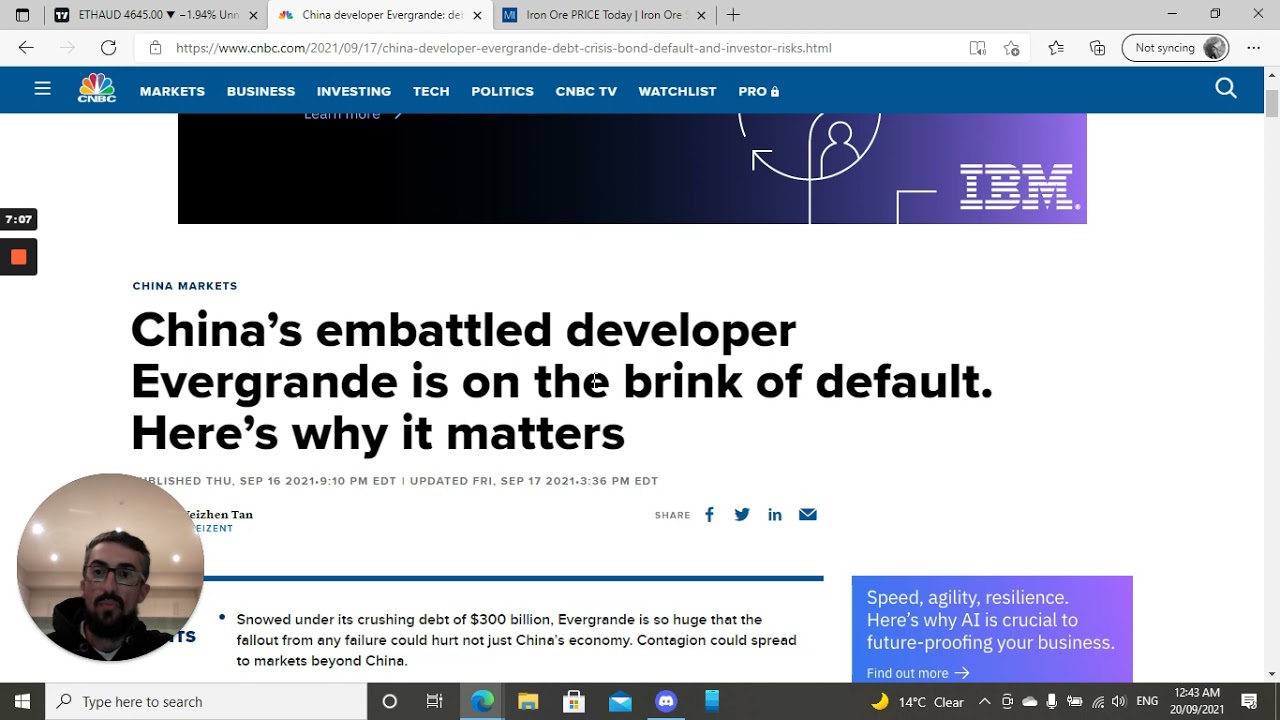The image is a screenshot of a CNBC webpage featuring an article about China’s market, specifically highlighting the financial troubles of the real estate developer, Evergrande. The headline reads, "China's embattled developer Evergrande is on the brink of default, here's why it matters." The article was originally published on Thursday, September 16th, 2021, at 9:10 PM and was updated on Friday, September 17th, 2021, at 3:36 PM. 

In the bottom left corner of the screen, there's a circular bubble, possibly indicating a live stream or a Skype call. Inside the bubble, there's an image of a man with a beard and glasses, both of which are brown. He is dressed in a black hoodie over a white shirt. 

Additionally, the CNBC page features an IBM advertisement at the top. Another ad, located lower on the page, promotes the importance of AI for business resilience with the tagline, "Speed, agility, resilience – here's why AI is crucial to your future-proofing your business." 

At the bottom of the screenshot, a taskbar or dock is visible, showing various apps installed on the user's computer. Social media icons for sharing the article on Facebook, Twitter, and Instagram, as well as a link for sharing via email, are aligned on the article page.